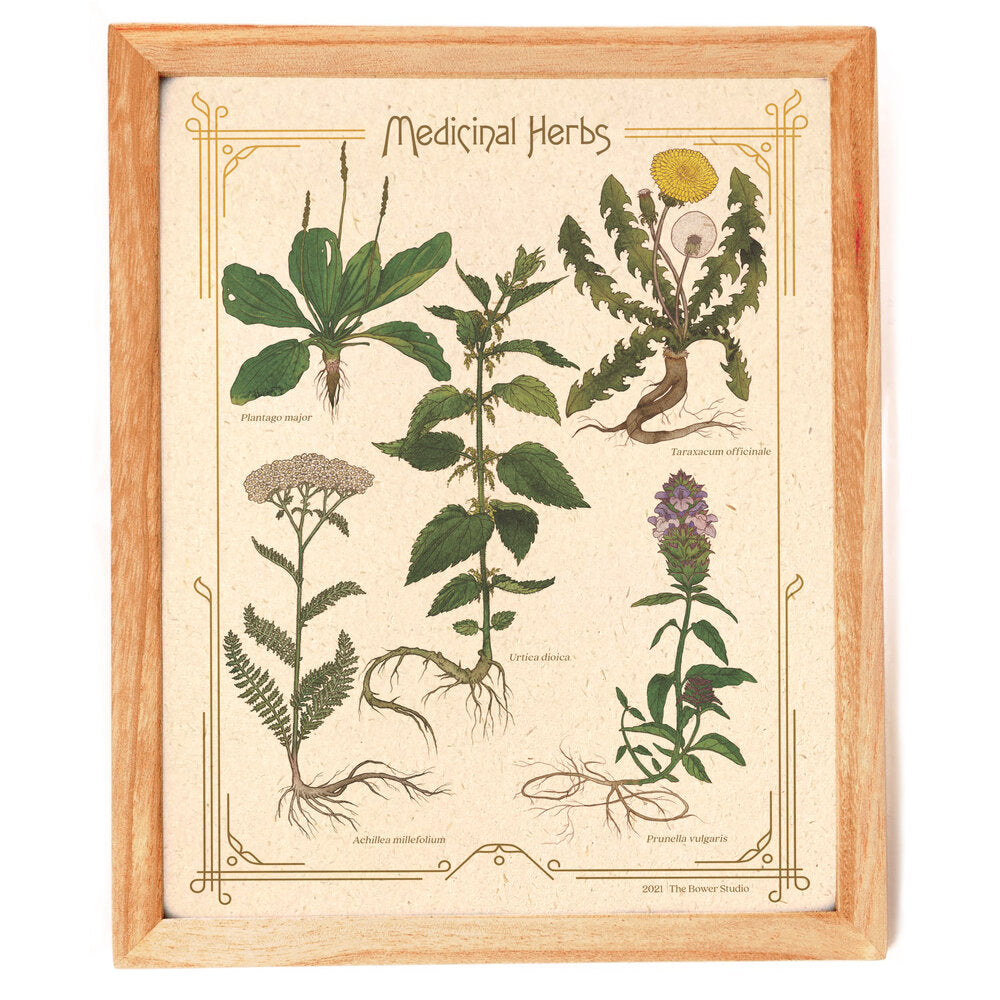The image showcases a finely detailed botanical illustration mounted in a wooden frame, prominently labeled "Medicinal Herbs" at the top. Within the frame, elegantly drawn plants are presented, each meticulously illustrating both the above-ground and root structures. The dandelion stands out with its bright yellow bloom and iconic globe of seed pods, while other plants, bearing various leaf shapes and small hairs on their roots, are also detailed. The illustration includes a plant with white flowers and fern-like leaves, another with purple flowers, and several others featuring distinctive leaf patterns and blooms. Although the Latin labels are illegible from a distance, the distinct characteristics of each plant are clearly depicted. The framed piece is bordered by an intricate line work design that shifts in color from dark brown at the bottom to a golden hue at the top, enhancing its visual appeal. The overall presentation elegantly marries artistic beauty with botanical accuracy.